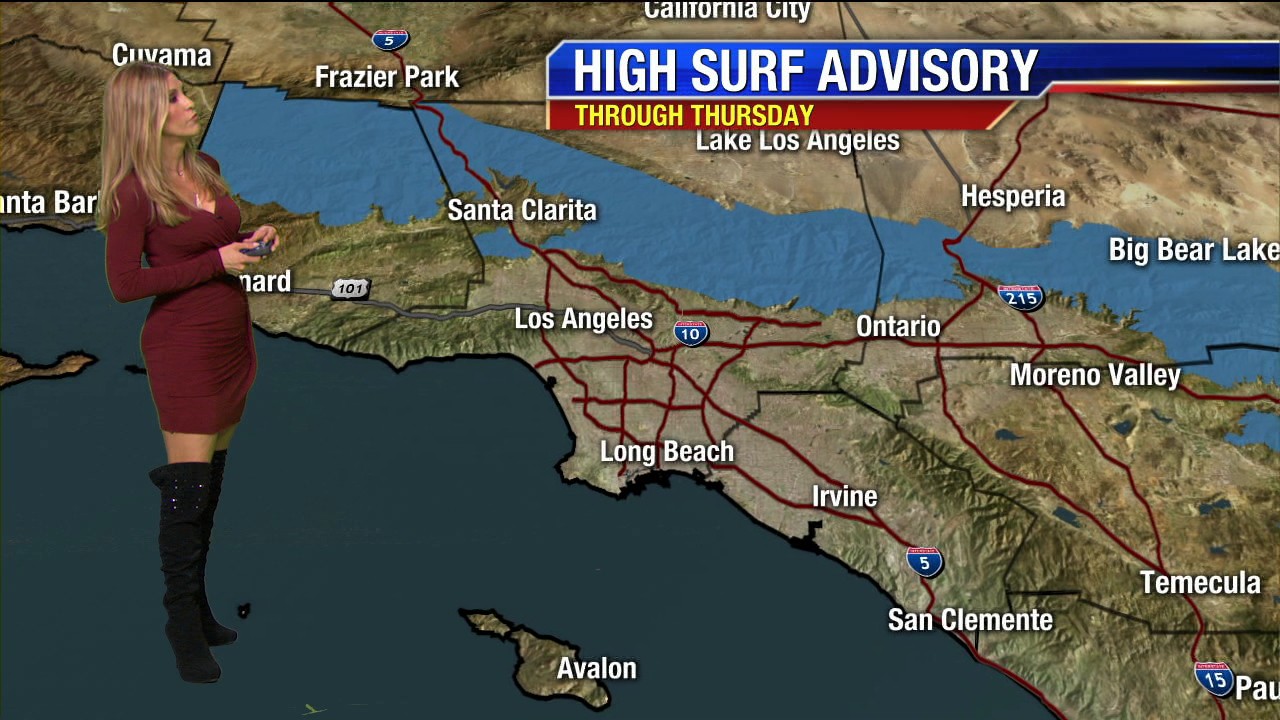The image depicts a weather report for Southern California, featuring a blonde female meteorologist in her 30s. She is positioned on the left side of the frame, facing right, and is dressed in a modern, tight-fitting maroon mini dress with black thigh-high boots. The background is a superimposed map highlighting a high surf advisory, with a gray-blue area representing water and a lighter blue channel. The map displays numerous locations including Los Angeles, Long Beach, Ontario, Irvine, San Clemente, Santa Clarita, Temecula, Moreno Valley, California City, Hesperia, Big Bear Lake, Lake Los Angeles, Fraser Park, Cuvamo, Santa Barbara, and Islet Avalon. Central to the visual is the high surf advisory, indicated by a blue bar with white text stating "High Surf Advisory" and a red bar below it with yellow text reading "Through Thursday."